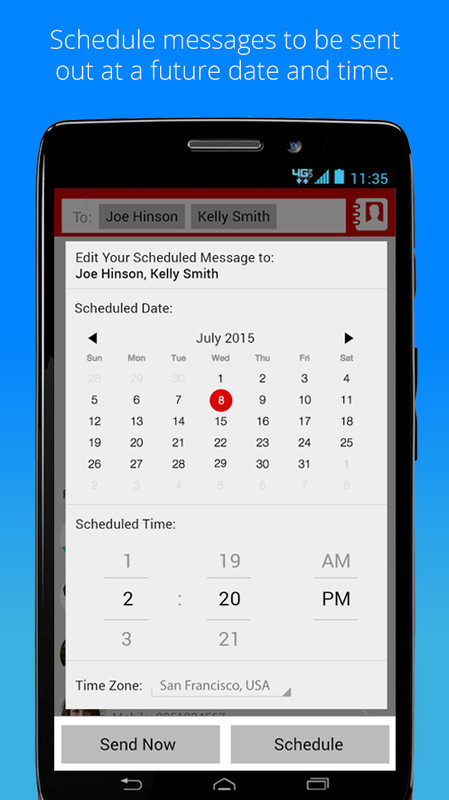This image is an advertisement screenshot for a scheduler or calendar app, set against a vibrant bright blue background. At the top, bold white text reads: "Schedule messages to be sent out at a future date and time." Below this text, the image features a smartphone, likely an Android device, possibly a Galaxy phone, with a black body. 

The app interface displayed on the phone screen shows a message scheduling feature, indicating recipients "Joe Henson" and "Kelly Smith." The editable message prompt states: "Edit your scheduled message to Joe Henson and Kelly Smith." Directly beneath the message text, users are presented with a calendar interface. 

The calendar is for July 2015, complete with left and right arrows to navigate between months. The user has selected July 8th, highlighted with a red circle. Beneath the calendar, there are scrollers to set the time, am or pm, and the time zone, which is set to "San Francisco, USA." 

At the bottom of the app interface, two buttons are visible. One reads "Send Now," and the other "Schedule," both featuring a gray background with black text. The phone interface also shows typical navigation buttons for return, home, and tabs. 

At the very top of the phone screen, icons indicate a 4G network with full five bars of signal strength, a fully charged battery, and the current time, which is 11:35. Additionally, the selfie camera icon appears above the 4G indicator, signifying the option for front camera use.